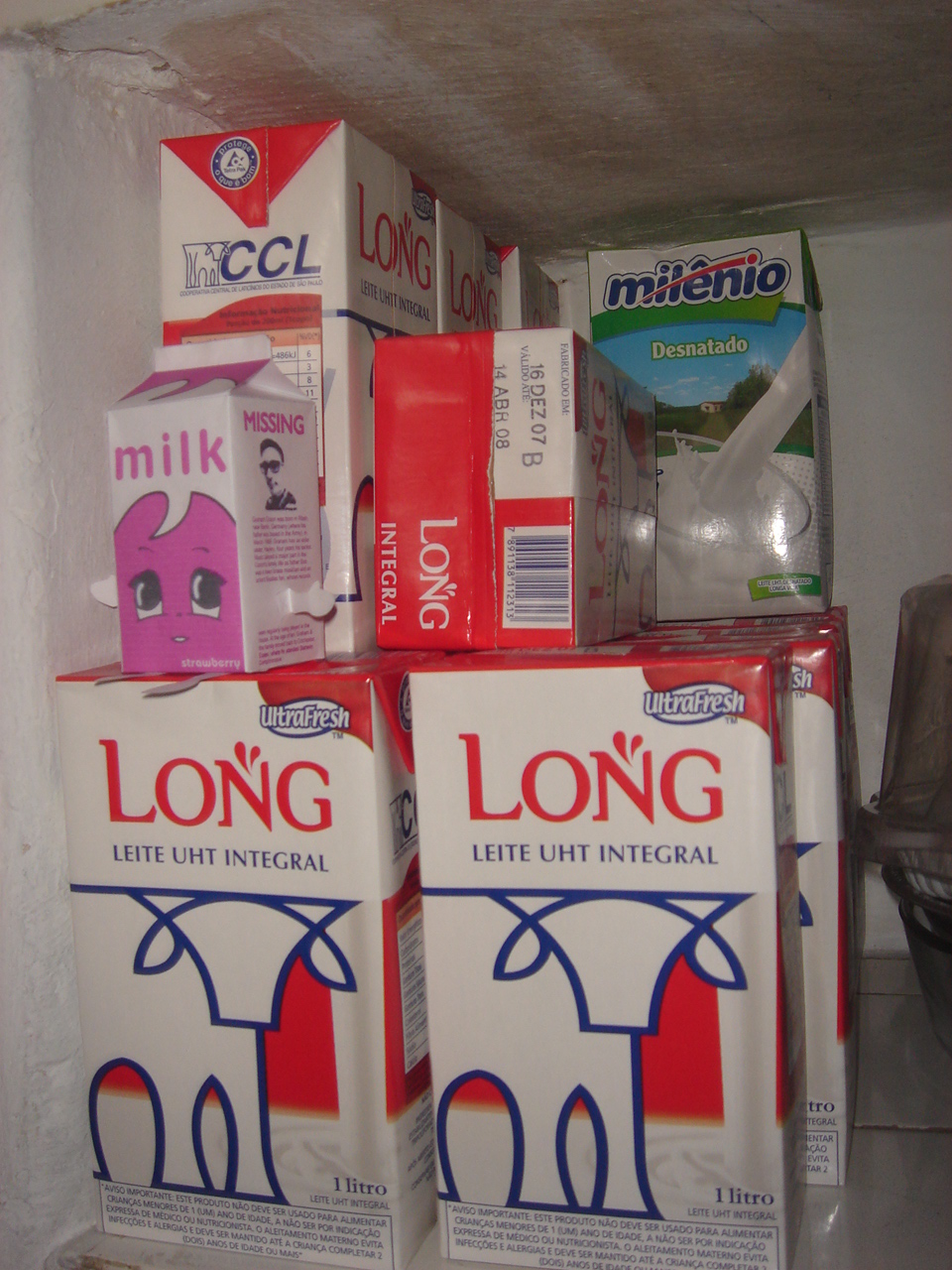The image features a stack of milk cartons neatly arranged on a shelf in what appears to be a storage room with unfinished drywall and ceiling. Most of the cartons are from the brand "Ultra Fresh" and prominently display the label "Long Latte UHT Integral," suggesting they are long-life milk products, likely in Spanish. These cartons, colored in red and white, also feature a drawing of a cow. Among them, there's a smaller, distinct milk carton with a white background and a playful cartoon face in pink, simply labeled "milk." Additionally, a carton labeled "Millennial" (or "M-I-L-E circumflex, M-I-O") and "Desnatado" sits towards the back, indicating it's a skim milk variant. There is also a mention of containers labeled "CCL" with glass illustrations. The overall scene, captured with a slight underexposure, shows a mix of carton sizes and designs, emphasizing the variety of milk products stored together.